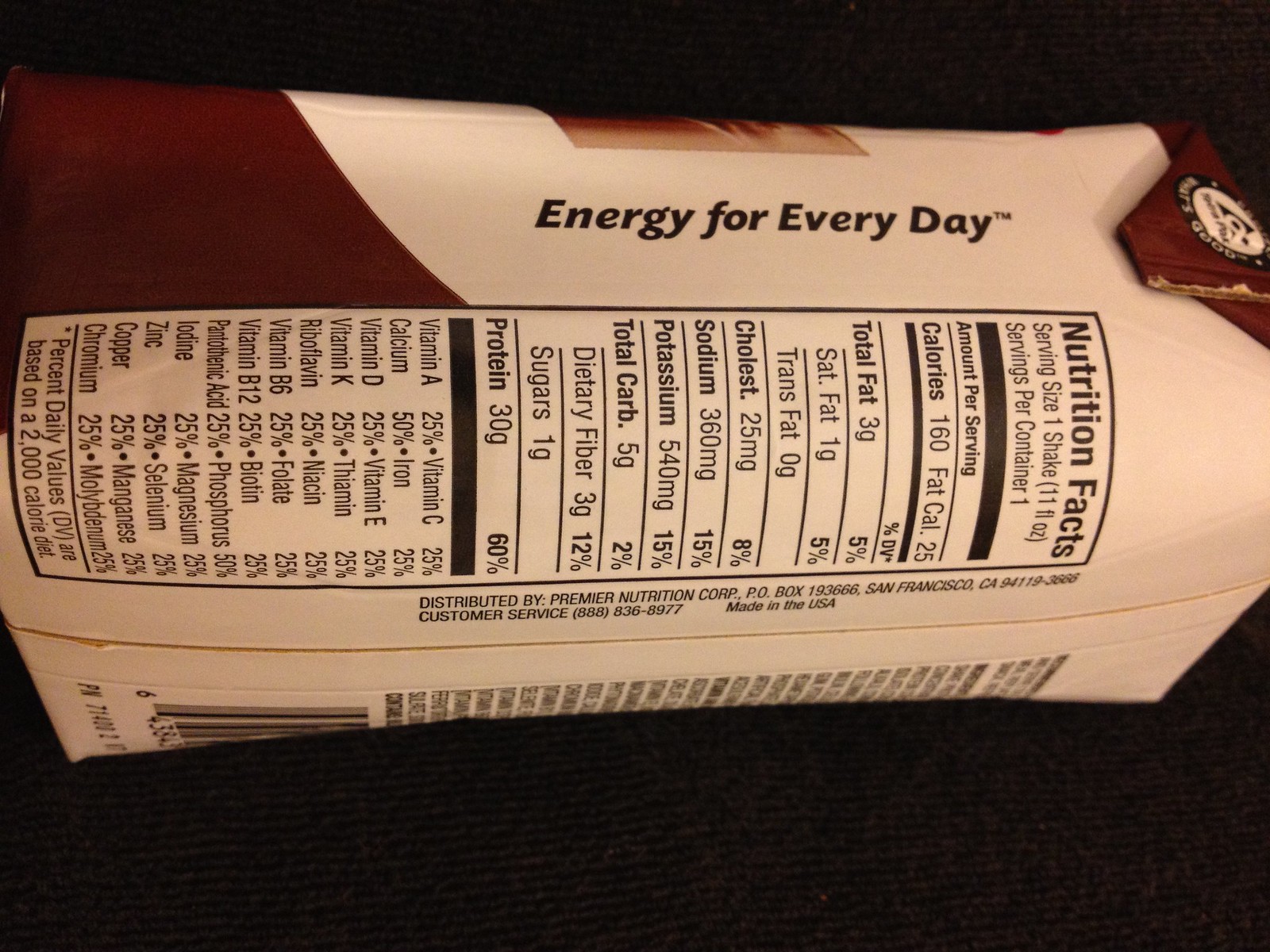The image is a detailed color photograph of a shelf-stable, ready-to-drink nutritional shake carton, lying on its side on what appears to be a black surface. The carton features a light pink and maroon color scheme with the text "Energy for Every Day" prominently displayed along with a trademark symbol. The side panel of the carton showcases the nutrition facts, revealing that the serving size is one shake, equating to 11 fluid ounces. Key nutritional information includes 160 calories, 3 grams of total fat (with 1 gram of saturated fat), 25 milligrams of cholesterol, 360 milligrams of sodium, 540 milligrams of potassium, 5 grams of total carbohydrates (comprising 3 grams of dietary fiber and 1 gram of sugar), and a substantial 30 grams of protein. The shake is enriched with various vitamins and minerals, providing 25% of the daily recommended intake for numerous nutrients like vitamin A, calcium, vitamin D, vitamin K, riboflavin, vitamin B6, vitamin B12, pantothenic acid, and iodine, based on a 2,000 calorie diet.